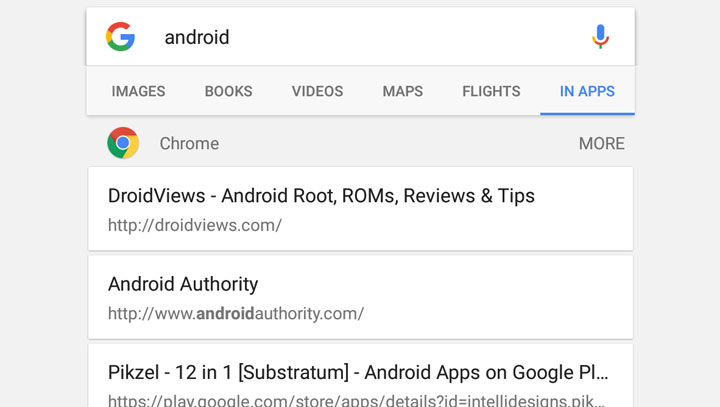This image is a screenshot from a Google app, likely captured from a tablet. The interface displays a Google search bar at the top, bearing the Google "G" logo on the left and the Google Assistant microphone icon on the right. The search term "Android" has been entered into the search bar. Below the search bar, there are several clickable tabs for different types of searches such as Images, Books, Videos, Maps, Flights, and Apps. The "Apps" tab, which is highlighted in blue indicating it is selected, is the last tab on the right. 

Underneath the tabs, there is an indication that the search results will open in the Google Chrome browser, marked by the Chrome logo and the word "Chrome." The first search result is titled "Droid Views, Android root ROMs, reviews and tips" from the website droidviews.com. The second result is from "Android Authority" available at www.androidauthority.com. The third result showcases an app named "Pixel (P-I-K-Z-E-L) 12-in-1 Substratum" available on the Google Play Store, and it includes a direct link to the Play Store.